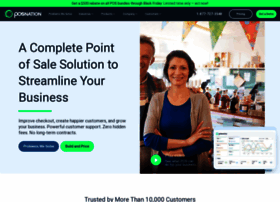The image appears to be a slightly blurry screenshot of a webpage, possibly advertising a point of sale (POS) system for businesses. The key elements of the image are as follows:

At the center-right of the image, there's a navy blue text that reads, "A complete point of sale solution to streamline your business."

Below this text, there are two buttons. The first button is blue, located towards the bottom left corner, and the second button is green, situated to the right of the blue button.

On the right side of the image, there's a picture of a woman wearing a blue t-shirt with some brown details. Behind her stands a man, though details about him are minimal because of the blurriness. A play button is visible in the bottom right corner of this picture.

Towards the bottom right of the webpage, there is a blurry line graph, indicating some form of data visualization or performance metrics.

At the bottom of the image, text reads, "Trusted by more than 10,000 companies" or "10,000 customers."

The top part of the image, which seems to be the header of the webpage, has various tabs, although they are indistinct due to the blurriness. The background color of the tabs is dark blue.

On the top right corner, there are two buttons—one green and one dark blue. 

In the top left corner, the name of the webpage is displayed in white text. The icon is green and starts with the letters "P" and "O," but the rest of the text is indistinct due to the blurriness.